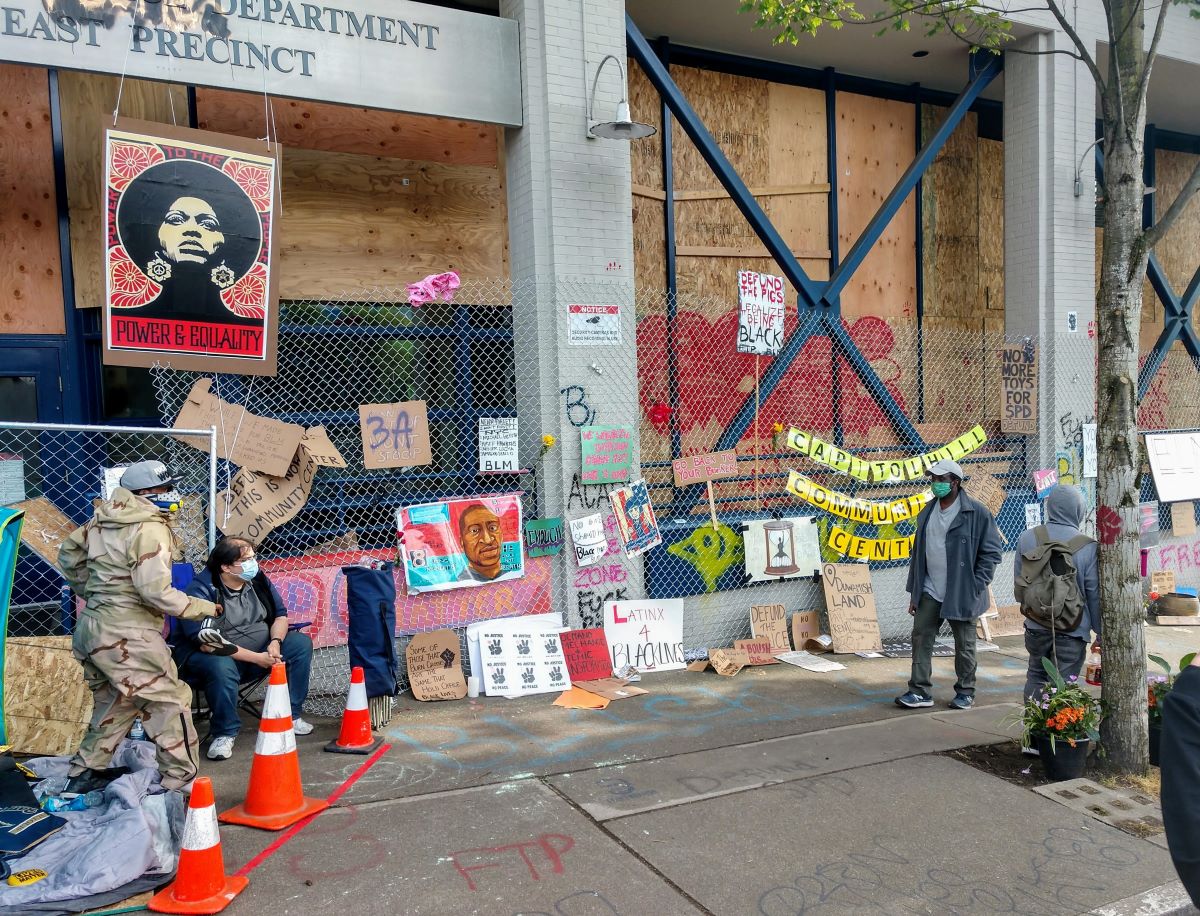The image depicts a scene in front of a police department that appears to be heavily fortified and closed off, with the building boarded up and surrounded by a chain-link fence. The fence is adorned with numerous posters, signs, and images related to the Black Lives Matter movement. Prominently displayed is a red and black artist's rendering of a Black woman with a round afro, reminiscent of the Obama Hope poster, which includes the words "Power and Equality" at the bottom. Another notable image displayed on the fence is a cartoon-like drawing of George Floyd.

The background structure is further secured with barbed wire and metal frames forming an X between concrete pillars. Part of a sign indicating "Department East precinct" in blue text on a gray board is visible.

In the foreground, several people, all wearing face masks, are seen gathered, suggesting a protest. Among them are two African-Americans and one white male. One person is wearing camouflage clothing, a mask, and a baseball cap. Bright orange cones with white rims are positioned on the left side of the image, along with graffiti adorning the concrete sidewalk. Additionally, yellow cards with black letters spell out "Capitol Hill Community Center" on the chain-link fence. Other details include various posters and a tree on the right side of the image.